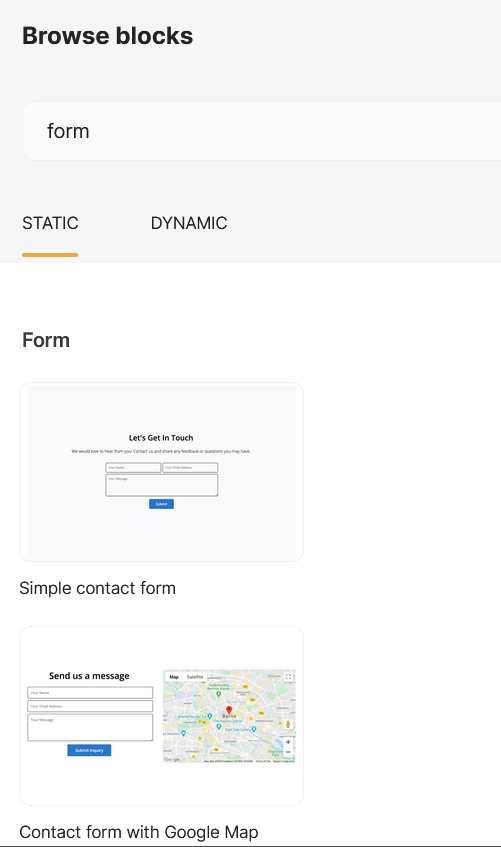This screenshot captures a section of a web page or software application, meticulously cropped to exclude any revealing brand markings, navigation menus, or web browser details. At the top of the image, the header "Browse Blocks" is prominently displayed in black text. Directly beneath this, a white search bar shows the search term "Form" entered into it.

Below the search bar, there are two navigational buttons labeled "Static" and "Dynamic." The "Static" button is selected, which is visually emphasized by an orange bold line beneath it. The search results for "Form" are displayed below these buttons.

The first search result features a straightforward contact form designed for website building, consisting of two smaller input fields and one larger text input area. The second search result is a contact form integrated with Google Maps. This layout includes a simple three-field input area accompanied by a live Google Maps image on the right-hand side. The screenshot doesn't include other options or results that might be available on the page.